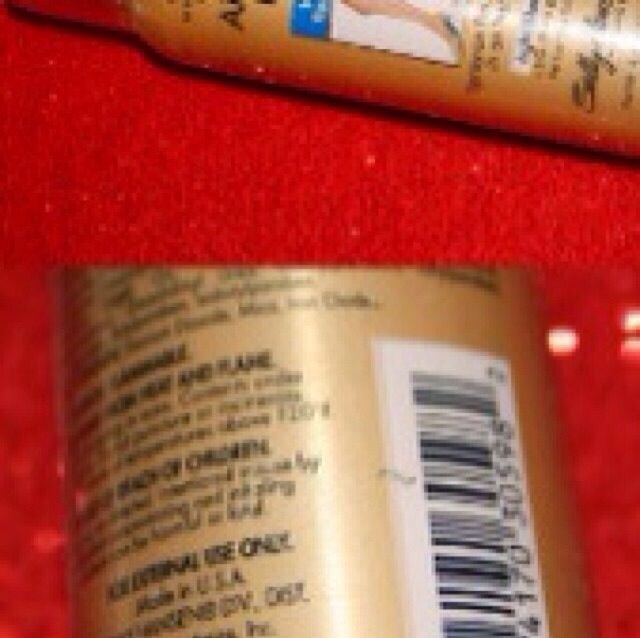This image features a dual-pane, horizontally split composition of a gold plastic bottle. The upper pane displays the bottle at a horizontal, slightly skewed angle, with the golden surface reflecting light. Despite the blurriness, one can discern that the bottle is adorned with black lettering and a white label depicting a woman's leg. The text on the top pane is not legible due to the lack of focus. In the lower pane, the bottle is shown in closer detail, making some of the text clearer. The words "FLAME," "HEAT," and "FOR INTERNAL USE ONLY" can be seen, along with the phrases "MADE IN USA" and a visible barcode. The gold bottle's shiny surface continues to reflect light, adding a gleam that accentuates its metallic appearance.